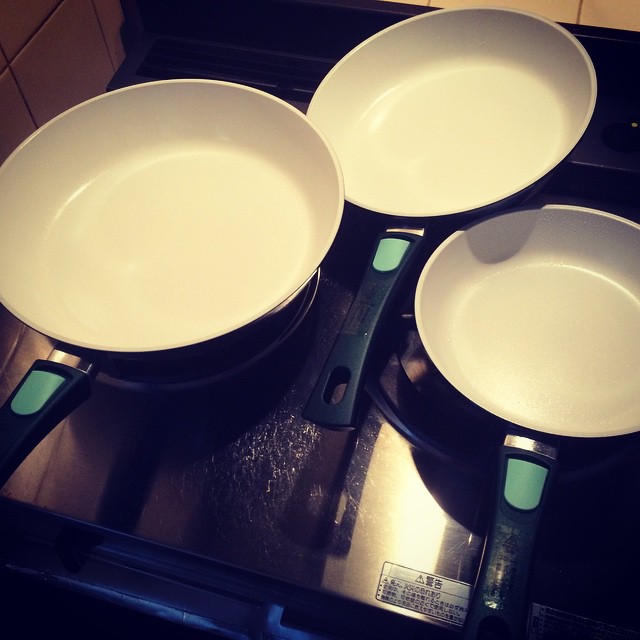The image showcases a set of three pristine, nonstick Teflon frying pans in varying sizes, arranged on a silver flat stove with a black surface. Each pan features a black handle accented with a small rounded light green shape near the attachment point. The interiors of the pans are a clean, unused white, contrasting with the black and green exteriors. One pan is positioned in the upper right middle of the frame, while the other two are below it. A small white sticker with Asian characters is visible on the bottom right corner of the stove. The scene is a bird's-eye view with a background of beige square tiles, indicating the pans are situated in the corner of the kitchen. The handles of the pans have holes at their ends, and one handle has a transparent sticker.